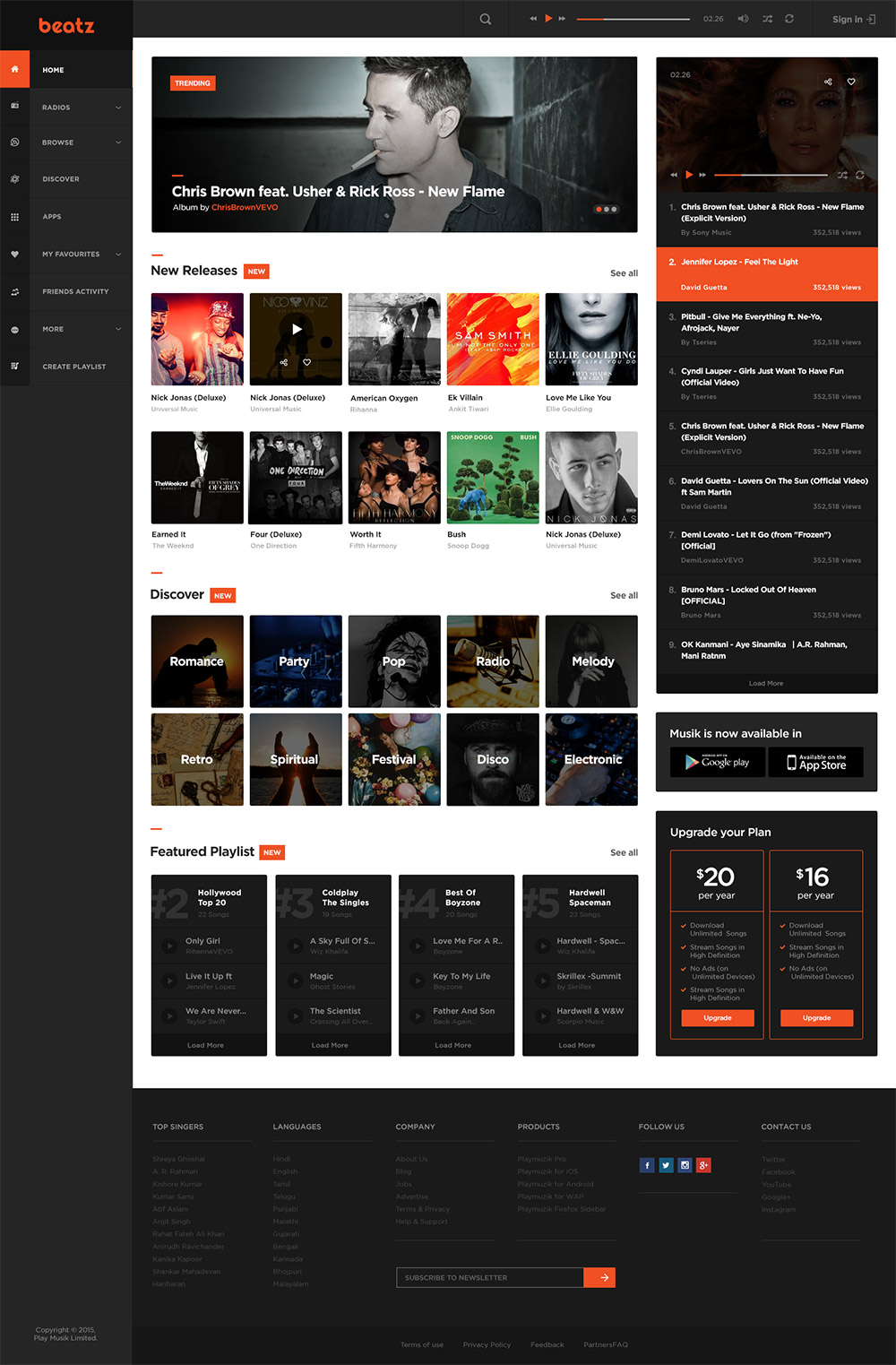The image showcases a music streaming platform called "BEATZ" with a sleek black vertical menu on the left-hand side. The menu, highlighted in orange, lists the following options: Home, Radios, Browse, Discover, Apps, My Favorites, Friend Activities, More, and Create Playlist. 

To the right, the user interface shifts to a white background with a New Releases section prominently displayed. Featured albums and singles include "Nick Jonas Deluxe" (repeated multiple times), "American Oxygen" by K-Villain, "Love Me Like You Do," "Earned It" by The Weeknd, "Four" by One Direction, "Worth It" by Fifth Harmony, and "Bush" by Snoop Dogg.

At the top of this section, there is a banner image highlighting trending artists such as Chris Brown, Future, Usher, and Rick Ross with the song "New Flame." Below this banner, there is a Discover category section featuring various genres and moods, such as Romance, Party, Pop, Radio, Melody, Retro, Spiritual, Festival, Disco, and Electronic.

On the far right, the currently playing song is "Feel the Light" by Jennifer Lopez. Additionally, there is an option to upgrade the subscription plan with two highlighted choices: $20 per year or $16 per year.